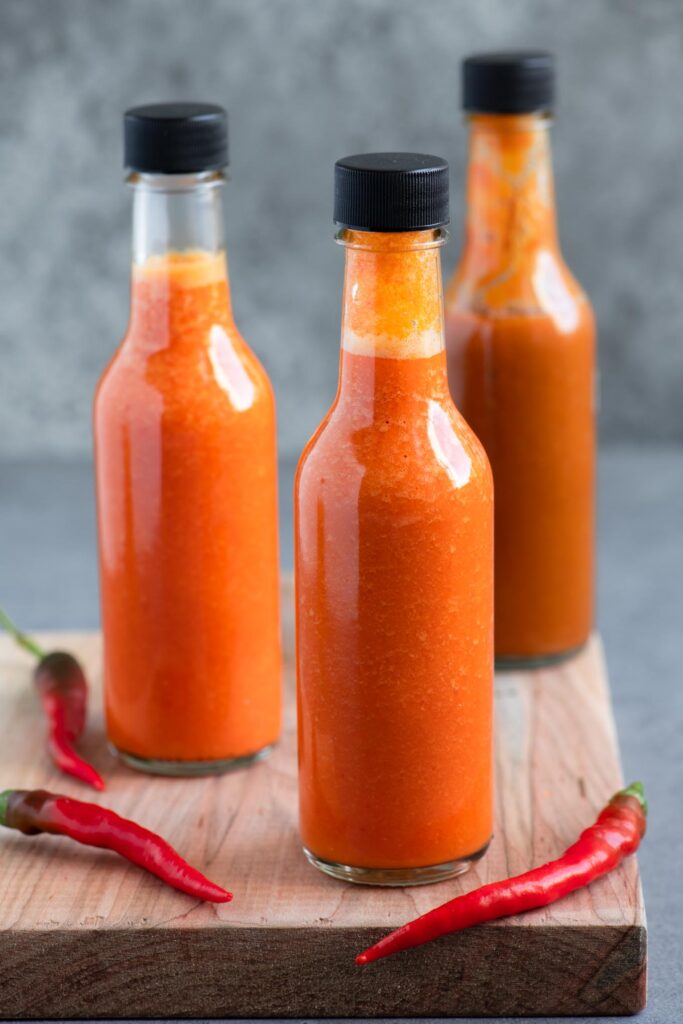This vertically-oriented rectangular image showcases a close-up view of a natural light wood butcher block table. Centered on the table are three identical glass bottles, reminiscent of classic Coke bottles, each filled to the brim with a vibrant orange sauce that suggests it might be hot sauce. The bottles are uniformly topped with black caps. Below them, three long, glossy red chili peppers are aligned, adding a touch of vivid red to the composition. The background is an out-of-focus gray, providing a neutral backdrop that accentuates the details in the foreground. A soft light from the right side highlights each bottle, casting subtle reflections on their surfaces.